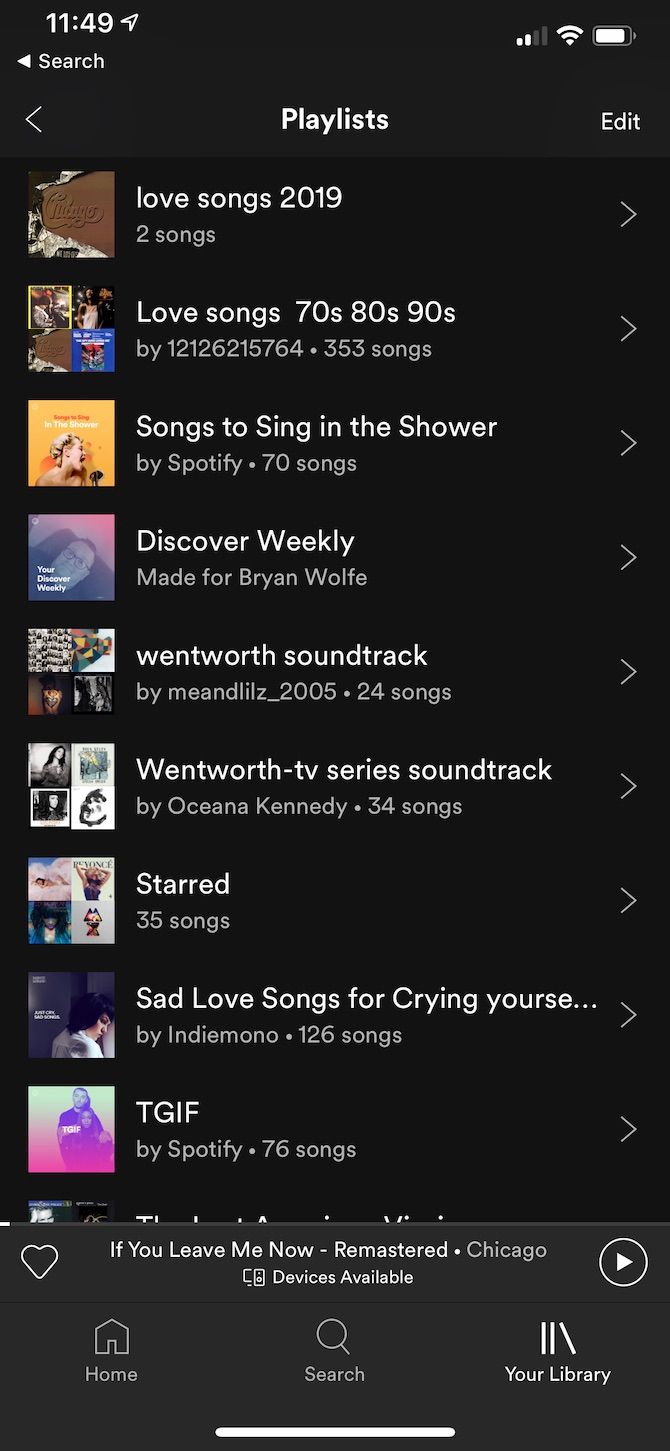The image is a screenshot of a music app on someone's phone displaying their playlists. The background is black with white text. At the top left of the screen, the time is shown as 11:49 alongside a location symbol. On the top right, the service bars are indicated with two bars lit, a full Wi-Fi signal, and an almost full battery icon.

Below the top bar, the word "Playlists" is prominently displayed. The screen shows a total of nine playlists:

1. **Love Songs 2019** - 2 songs
2. **Love Songs 70s, 80s, and 90s** - 353 songs
3. **Songs to Sing in the Shower** - 70 songs
4. **Discover Weekly** (made for Brian Wolfe) - Wolfe spelled as B-R-Y-A-N and W-O-L-F-E
5. **Wentworth Soundtrack** - 24 songs
6. **Wentworth-TV Series Soundtrack** - 34 songs
7. **Starred** - 35 songs
8. **Sad Love Songs for Crying Yourself...** - 126 songs
9. **TGIF** - 76 songs

At the bottom of the screen, the currently playing song "If You Leave Me Now (Remastered)" by Chicago is shown, accompanied by a play button and an unlit heart icon indicating the song is not marked as a favorite. There's a note saying "Device is available". At the very bottom of the screen are the navigation buttons: Home, Search, and Your Library.